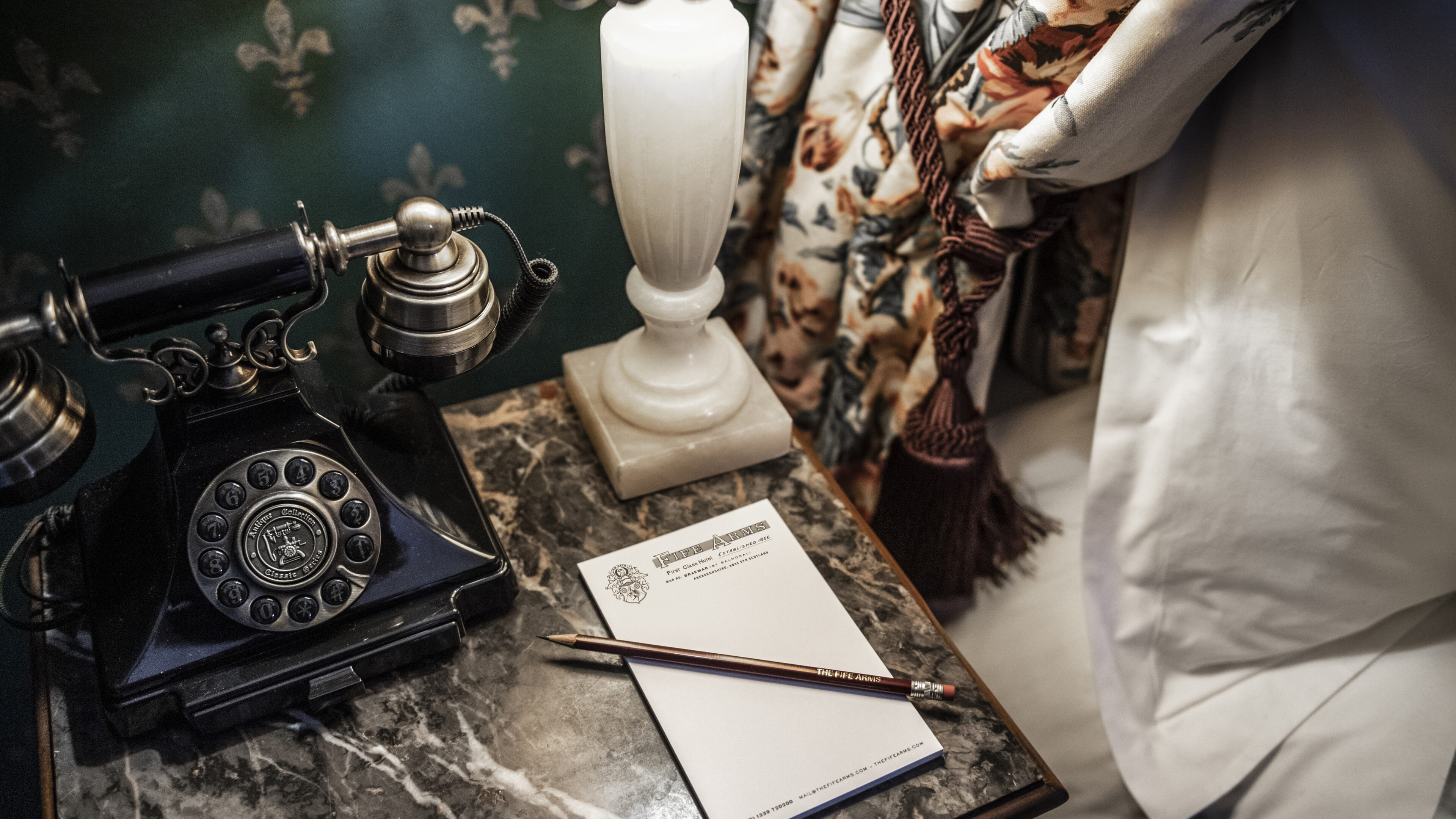The image captures a vintage scene centered around a black rotary phone with chrome handles, likely from the 1930s, resting on a beautifully patterned marble table. The table's surface showcases a mix of black, white, and brown hues, enhancing the elegant, historic ambiance. Adjacent to the phone, a small pad of paper sits with a pencil laid diagonally across it, the paper possibly bearing an emblem and tiny lettering that suggest a hotel name and location. Behind this arrangement, a white marble lamp base adds a touch of sophistication, while the background features a dark or blue wallpaper with designs, contributing to the classic look.

To the right of the phone and notepad, a heavy drape adorned with a floral pattern and held back by a thick, copper-colored rope tassel frames the scene, adding depth and texture. The bed is partially visible to the right, with pristine white pillows and sheets providing a stark contrast to the rich, detailed elements on the marble table. Overall, the photograph exudes a timeless elegance, merging vintage details with a refined setting.